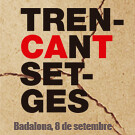This is a small photograph, roughly the size of three or four postage stamps, featuring a detailed inscription on a tan, cracked plaster wall. The image displays bold, capitalized letters in distinct lines. The first line spells "T-R-E-N-" in black, followed by "C-A" in red and "N-T" in black on the second line. The third line reads "S-E-T-" in black, with the final line "G-E-S" also in black. At the bottom, the text reads, "BOTELINA, 8 DE SETEMBRE," suggesting it is in another language. The crack on the wall is accentuated by three squiggly lines running through the image, hinting at a deeper context that may signify a historical or protest-related significance.